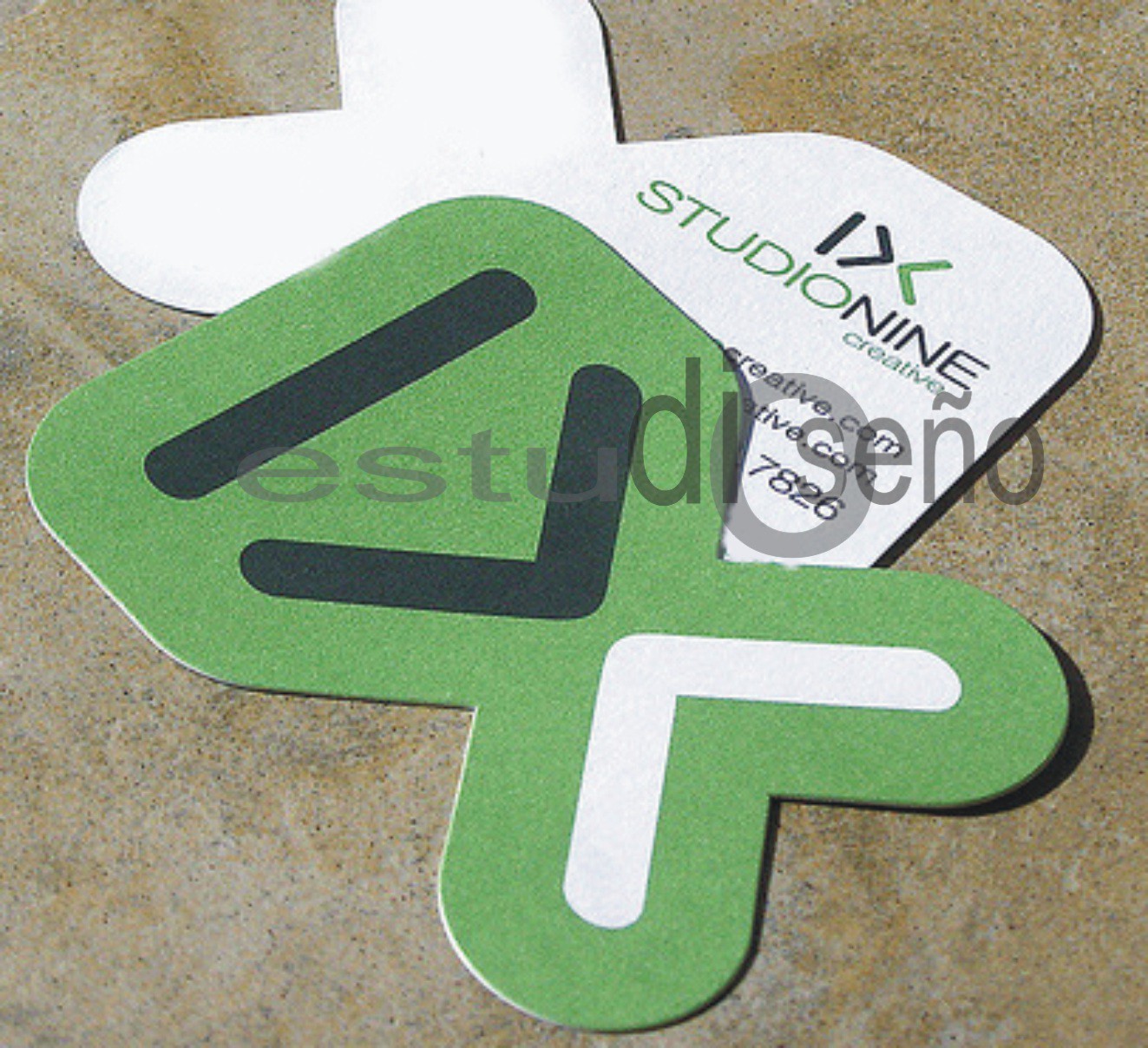The image captures two flat objects laying on a brownish, possibly concrete surface that has some discolored stains. These objects are similar in shape, appearing thin, and could be business cards, coasters, or mouse pads. One object shows the front side, while the other is turned over to reveal the back.

The object showcasing its front side is green with a distinct design: a straight black line across the flatter end, flanked by a black greater-than symbol and a white less-than symbol, creating a visual effect reminiscent of tail fins or a triangle with a pointed arrow pattern. The other object, showing its backside, is white with the following text partially visible: "Studio 9 Creative," "Creative.com," and a phone number ending in 7826. An additional watermark in semi-transparent gray text reading "Estudio Sino" appears across the center of the image, suggesting another layer of branding or design possibly in Spanish.